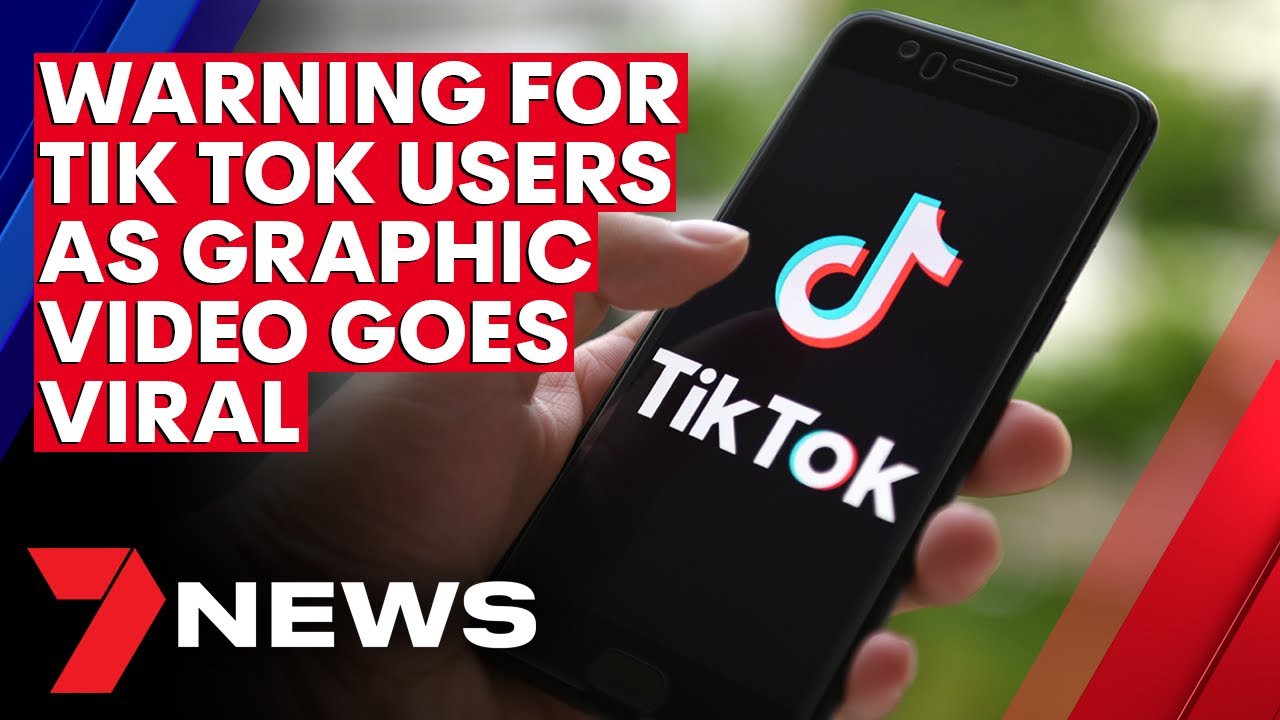The image appears to be a screenshot from a news website or possibly a thumbnail from an advertisement or YouTube video for an outlet called 7NEWS. The bottom left corner of the screen features a distinctive red logo resembling a folded ribbon or strip of paper shaped into the number 7, with the word "NEWS" in white capital letters beside it. In the main portion of the image, a white man's left hand is holding a black mobile phone displaying the TikTok app, identifiable by its recognizable logo: a stylized, 3D music note with a 70s retro aesthetic in blue, red, and white colors, accompanied by the text "TikTok" in white. Overlaid across the top of the image is a prominent red banner with white text that reads, "WARNING FOR TIKTOK USERS AS GRAPHIC VIRAL VIDEO GOES VIRAL." This suggests a cautionary message about a graphic video circulating on the TikTok platform.